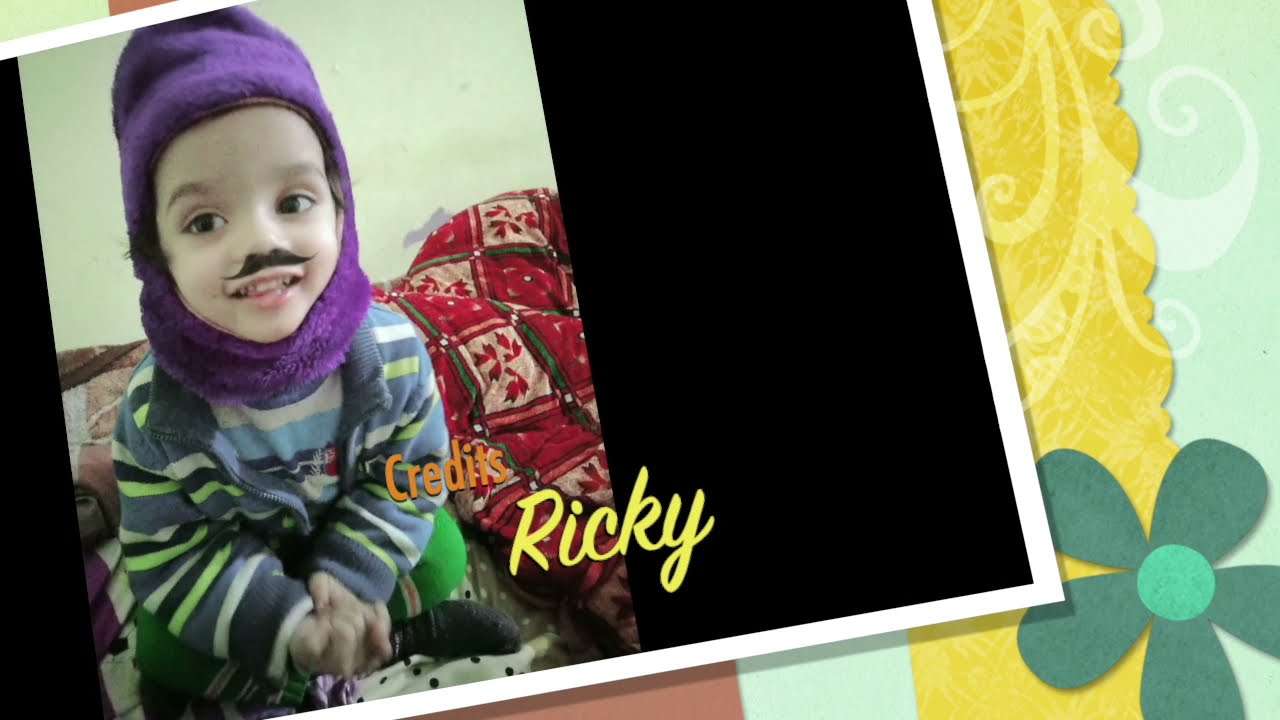The image is a detailed and vibrant collage resembling the front page of a picture book or a photo album. The main focus is an old-style Polaroid photo superimposed at an angle. Within the Polaroid, a young boy, possibly around two years old, sits, beaming in a playful costume. He wears a purple furry hat that encircles his face, much like a costume hood, paired with a matching purple furry collar around his neck. The boy's face features a pasted or drawn-on black mustache, adding to the whimsical nature of his attire. He dons a striped long-sleeved shirt in hues of green, gray, and blue. 

The background upon which the Polaroid rests is a layered paper craft with vibrant vertical stripes in red, light blue, and yellow. This background has textured shading, giving it a sense of depth. Additionally, a lineless teal flower with five petals and opaque white curls adds artistic flair to the backdrop. The right side of the Polaroid features a red and green blanket adorned with poinsettia or mistletoe designs, possibly indicating a festive Christmas setting. 

Above and in front of the Polaroid, in orange font, is the word "Credits," and in a yellow curly font, the name "Ricky" is prominently displayed.